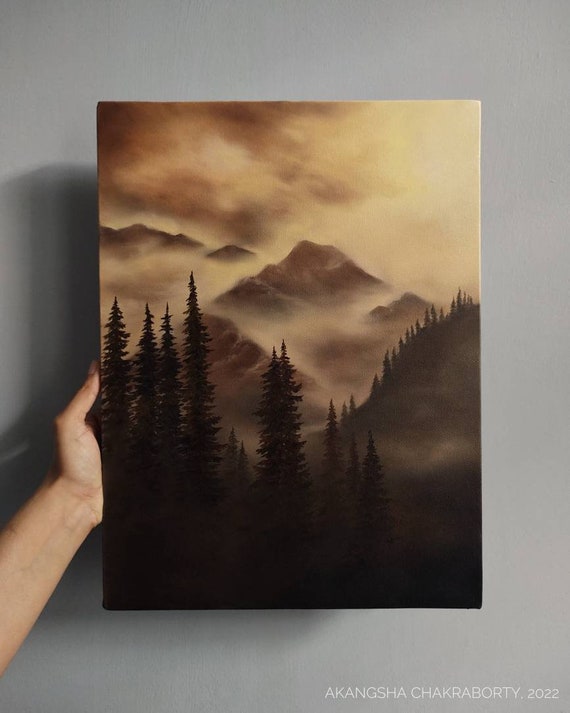In this bright, indoor photograph, a left-handed white person is holding up an oil painting on canvas against a light gray wall. The painting, signed "Akanksha Chakraborty, 2022" in the bottom right corner, captures a misty outdoor landscape. Dominated by dark, earthy tones such as black, brown, and forest green, the scene showcases a dense forest of silhouetted pine trees set against a backdrop of mist-covered mountains. The sky above is dramatic and varied; the top right corner glows with an orange hue, likely reflecting the setting sun, while the top left is overcast with dark clouds. The painting's overall ambiance is one of serene and moody natural beauty, intricately detailed in its depiction of trees, fog, and mountainous terrain.